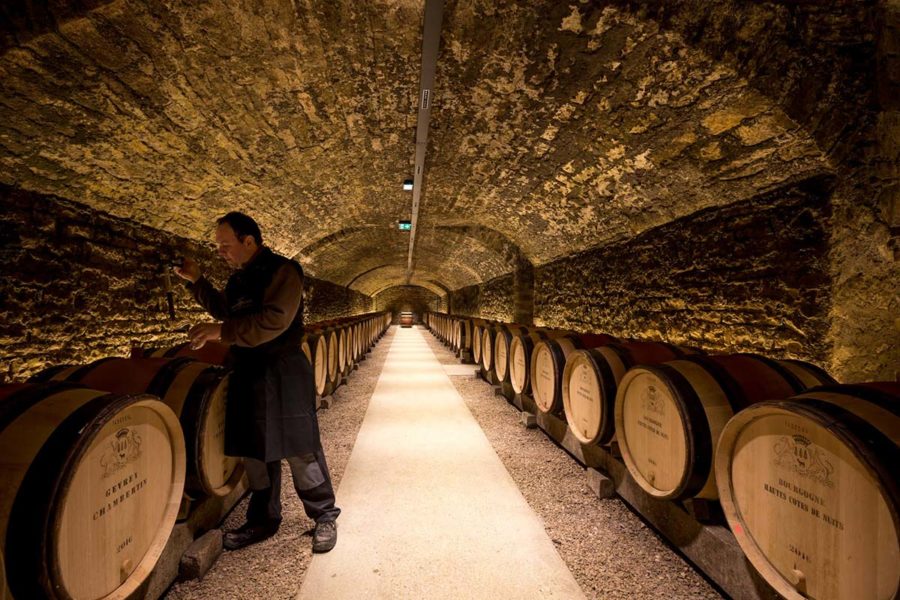The photograph captures the interior of a wine vault resembling a cave, with stone walls and a curved ceiling featuring a mix of dark and lighter tan patches. Lining both sides of the pebble gravel floor, which has a central cream-colored walkway, are rows of wooden casks adorned with emblems and illegible text, with one notably stamped "2016." The cylindrical barrels, which bear colors of brown, maroon, and black, are positioned horizontally. On the left side, a man in dark clothing, including a black apron, is seen taking a sample from one of the casks using a pipe. The man, with short black hair, stands attentively focused on his task in this atmospheric and dimly lit tunnel-like space.